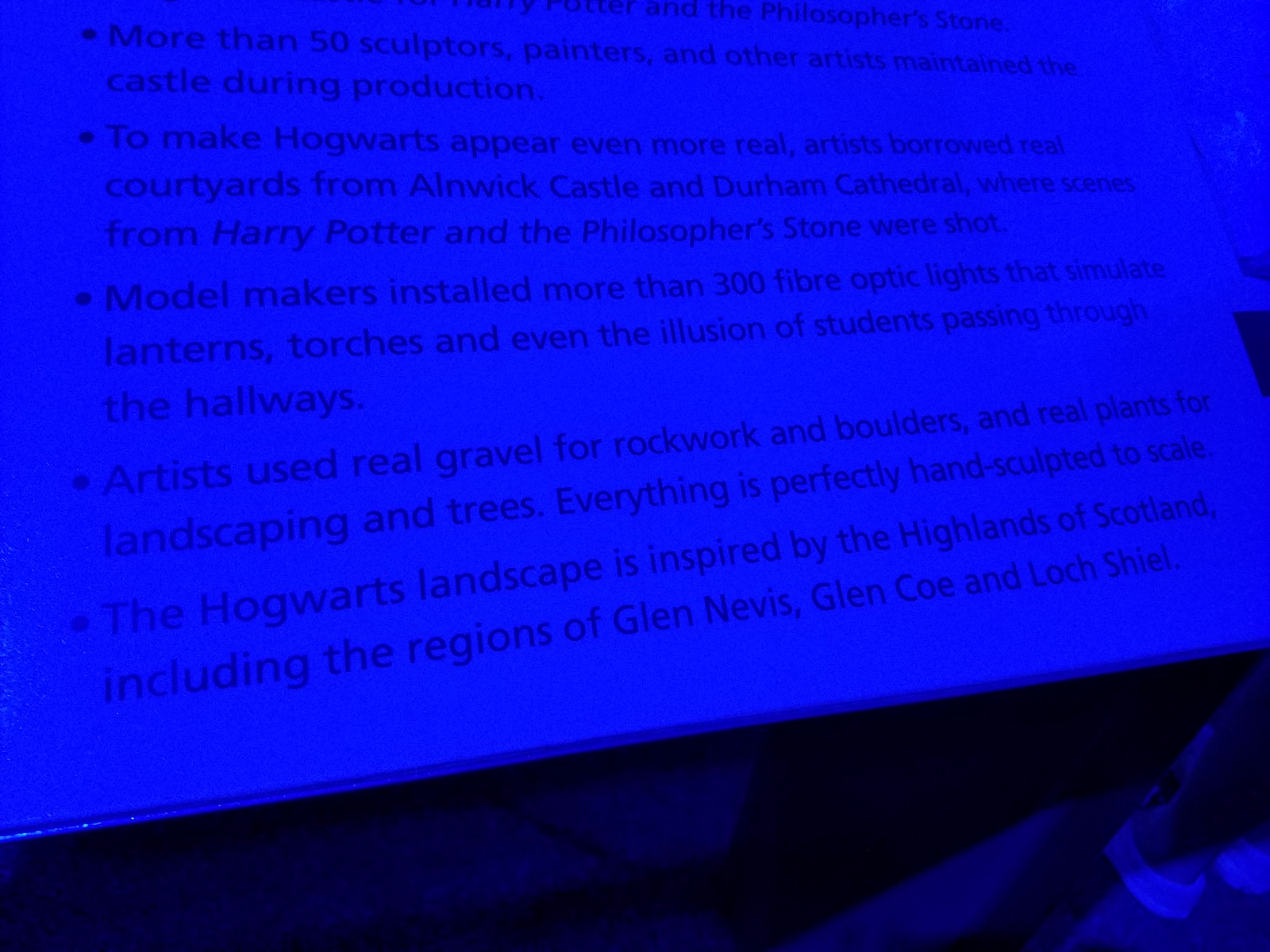The image captures a computer screen emphasizing a rich, dark blue hue, almost bordering on black in the lower regions, suggesting it was photographed in a dimly lit room. The screen, which seems to be slightly illuminated with a light electric blue background, displays text that is difficult to read due to the prevalent darkness. Nevertheless, discernible details reveal a series of bullet points related to the production of Hogwarts for the Harry Potter series. The highlighted points mention that over 50 artists, including sculptors and painters, maintained the castle during production. To enhance realism, artists borrowed elements from Alnwick Castle and Durham Cathedral, where scenes from Harry Potter and the Philosopher's Stone were filmed. Model makers installed more than 300 fiber-optic lights mimicking lanterns, torches, and student movement in the hallways. Real gravel, rock work, boulders, and plants were used, with all elements meticulously hand-sculpted to scale, and the Hogwarts landscape drew inspiration from Scotland's highlands, specifically Glen Nevis, Glen Coe, and Loch Shiel. The text appears to be printed on a sign that is slanted from the lower left to the upper right.